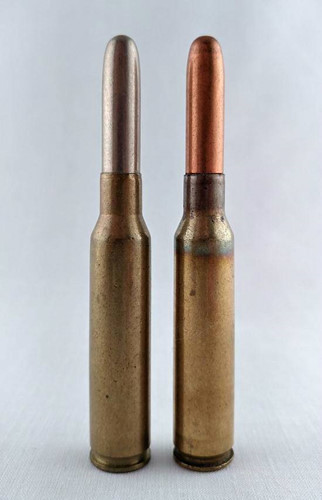A vertically aligned rectangular photograph features two tall, cylindrical objects that resemble bullets, positioned side by side. The background is a muted grayish-blue, almost smoky in appearance, which contrasts with the shiny, slightly rusty surfaces of the objects. Each bullet-like object has a brass body with narrow, elongated shapes. The left one has a shiny silver top, while the right one sports a reddish-brown, copper-colored top. They both have brown bases, with the metallic cylinders extending almost the entire length of the image, casting a subtle drop shadow. The photo captures the intricate details of the engravings and the textured, grainy surface they stand on, giving the image a sense of depth and age.